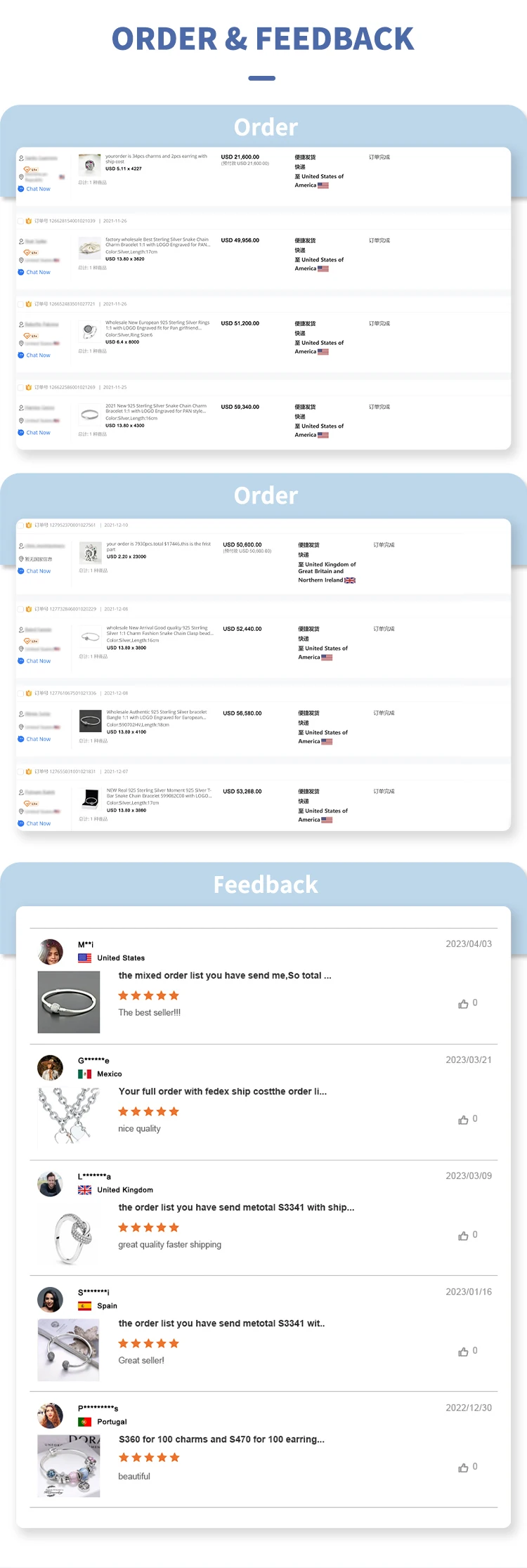The screenshot features a user interface composed of two main sections—'Order' and 'Feedback'—with a blue, almost periwinkle header. At the top, the highlighted section title 'Order and Feedback' is prominently displayed.

In the first 'Order' section, there are four choices each displayed with a small thumbnail image. The most prominent text within this section is the price of each item, making it easy to compare costs at a glance.

A second, nearly identical 'Order' section follows, also displaying four product choices with corresponding thumbnail images and bold prices.

Towards the bottom, the interface shifts to the 'Feedback' section, marked by a similar light blue banner. This section lists five different items, each accompanied by a brief description and a 5-star rating. All listed items appear to be jewelry and fashion accessories from various countries: the United States, Mexico, Spain, and Portugal.

The user interface efficiently combines the order options with detailed product feedback, streamlining the shopping experience for potential buyers.